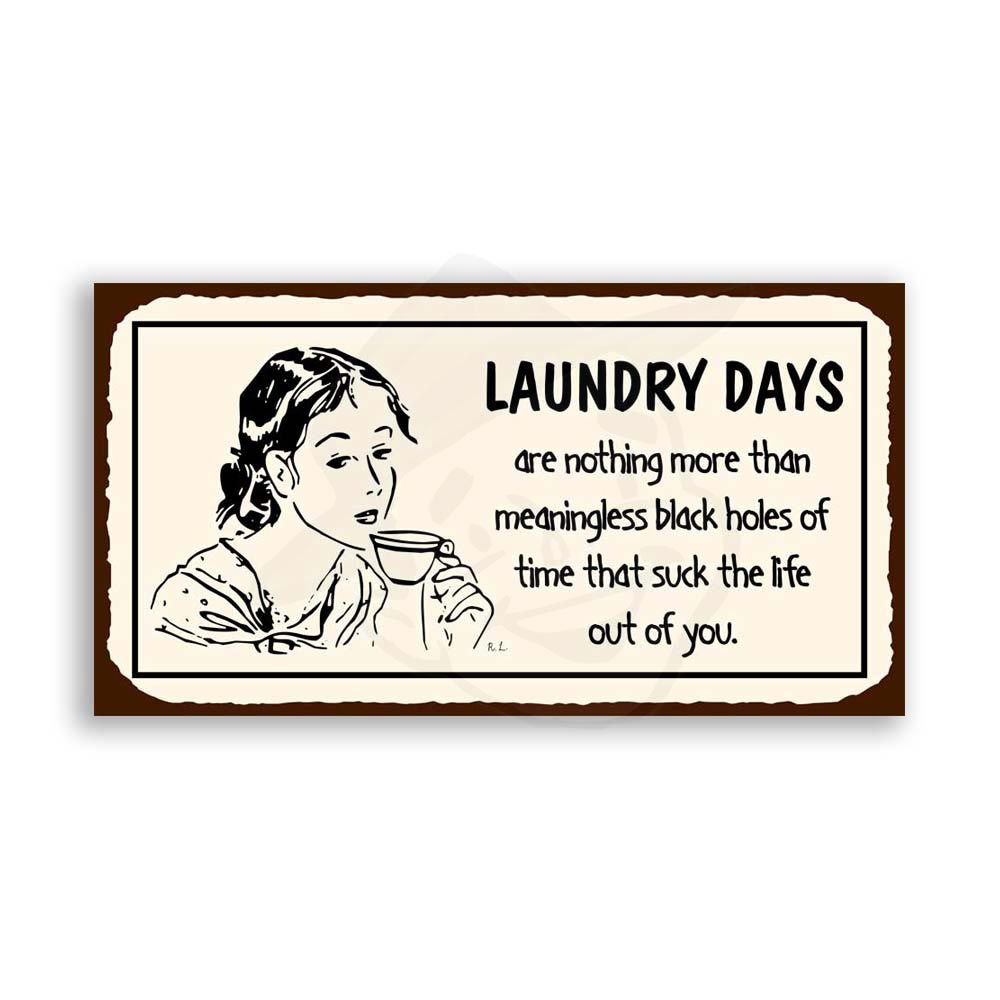The image depicts a modern yet vintage-styled rectangular sign designed to look aged, likely created using Photoshop or an art program. The sign features a dark brown border with a deckled edge, enhancing its old-timey appeal. Inside the border, an off-white rectangular area hosts the central elements of the design. On the left side, a detailed black-and-white ink drawing portrays a woman with her hair pulled back into a low bun, holding a small teacup up to her lips. She appears tired and contemplative, gazing downward toward the right of the image. To the right of the woman, bold black all-caps text reads "LAUNDRY DAYS," with a smaller, non-bold font underneath stating, "are nothing more than meaningless black holes of time that suck the life out of you." The text and the illustration are encapsulated in a rectangular box with a slightly jagged edge, giving it a decoupaged look. This whimsical and humorous placard, reminiscent of vintage signs, would be a charming addition to a laundry room or bathroom, or even a laundromat.